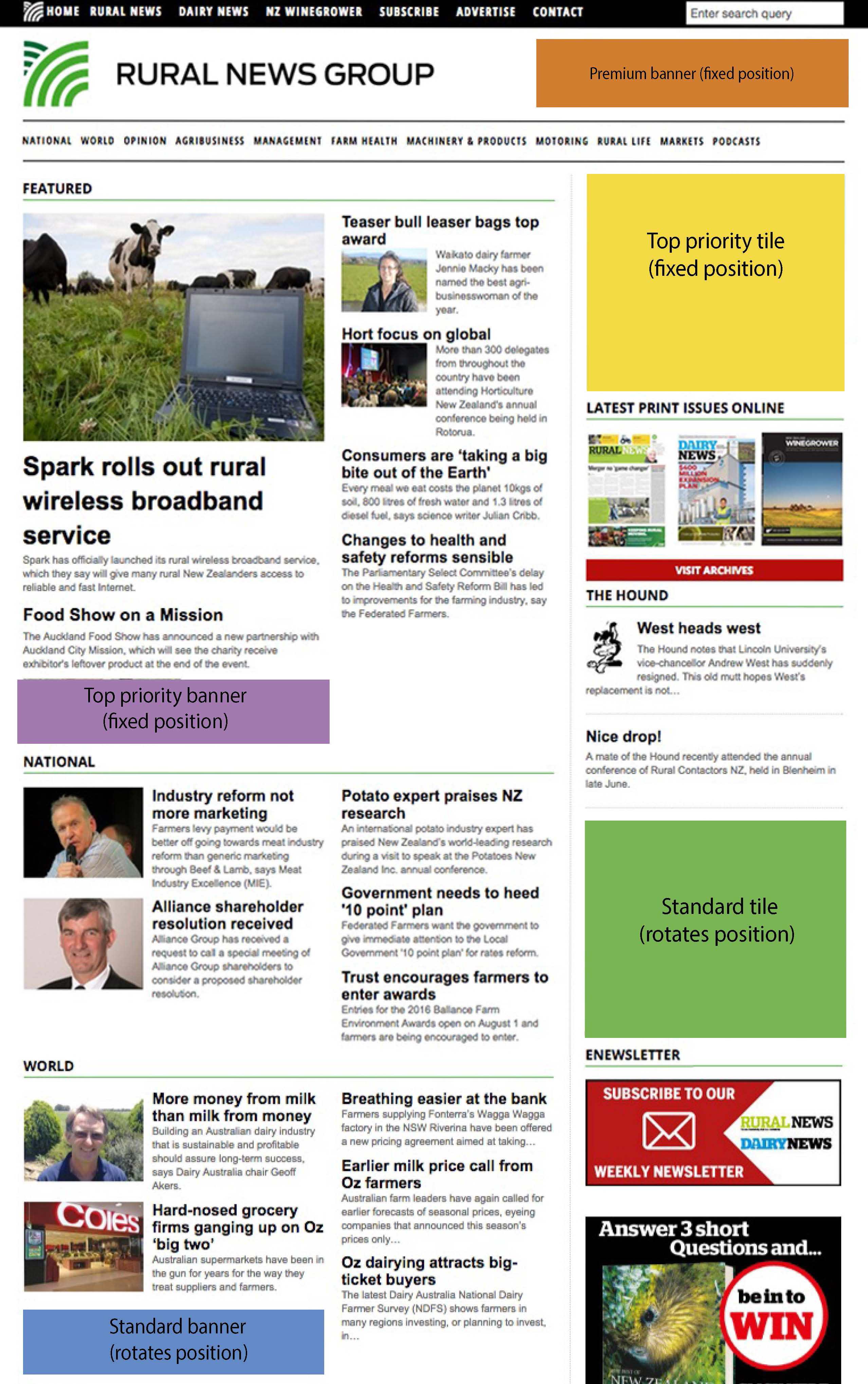**Detailed Caption for the Web Page Image**

The image depicts a comprehensive web page from "Rural News Group." The top of the page features a black banner with navigational tabs for *Home, Rural News, Daily News, NZ Wine Grower, Subscribe, Advertise, Contact*, and a search box. Below this banner is the company's logo, characterized by green arches, and the title "Rural News Group" prominently displayed. To the right of the title is a fixed position for a premium banner ad.

Further down, another set of tabs includes sections for *National, Rural, Opinion, Management, Farm Health, Machinery and Products, Motoring, Rural Life*, an unreadable category, and *Podcasts*. The main content area below these tabs showcases featured articles, with the leading headline being "Spark Rolls Out Rural Wireless Broadband Service." Surrounding this feature are additional articles: *Teaser Bull Razor Bags Top Award*, *Hort Focus on Global*, *Consumers Are Taking a Big Bite Out of the Earth*, and *Changes to Health and Safety Reforms*.

In the following sections, more articles are listed. Under *National News*, we see titles like *Industry Reform, Not More Marketing*, *Alliance Shareholder Resolution Received*, *Potato Expert Praises NZ Research*, *Government Needs to Head 'Ten Point' Plan*, and *Trust Encourages Farmers to Enter Awards*.

The *World News* section highlights five articles: *More Money From Milk Than Milk From Money*, *Hard Nosed Grocery Firms Hanging on OZ 'Big Two'*, *Breeding Easier at the Bank*, *Earlier Milk Price Call from OZ Farmers*, and *OZ Dairying Attracts Big Ticket Buyers*.

On the right side of the page, there's a segment for the *Latest Print Edition Online* and an invitation to subscribe to an e-newsletter. Additionally, users are prompted to answer three short questions for a chance to win a prize.